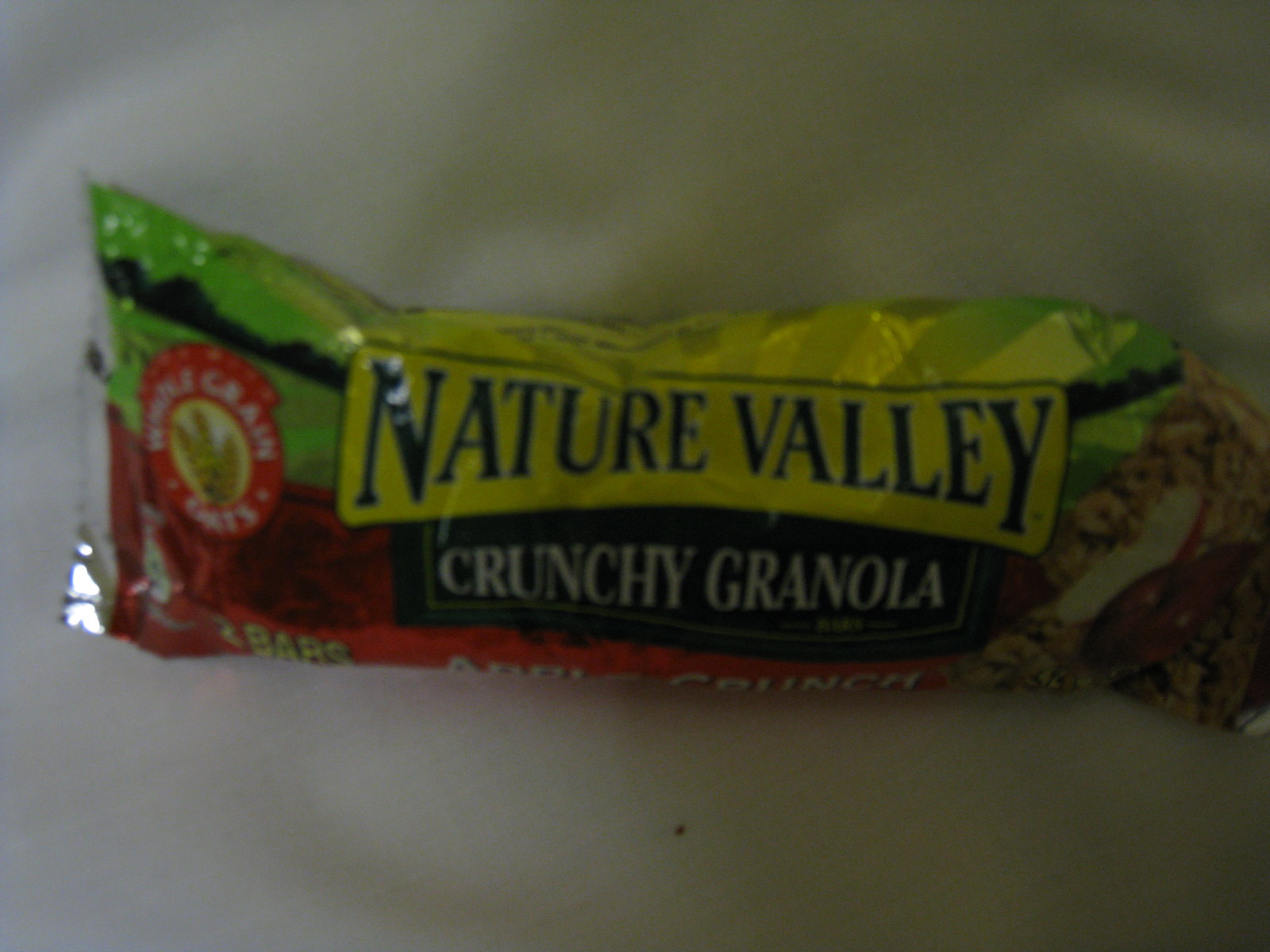This close-up image showcases a foil-wrapped granola bar package dominated by vibrant yellow, green, and red hues. At the center, the package prominently features "Crunchy Granola" text, while above it, the brand "Nature Valley" is clearly displayed. On the left side, there's a circular logo with a yellow wheat plant in its center, though the surrounding text is indistinct due to the proximity of the shot. The right side of the image reveals a textured granola surface, resembling light brown peanuts. The bottom edge of the package faintly reads "Apple Crunch," although the orientation makes it challenging to decipher. The overall ambiance of the image is dark and dim, suggesting an obscured light source above.